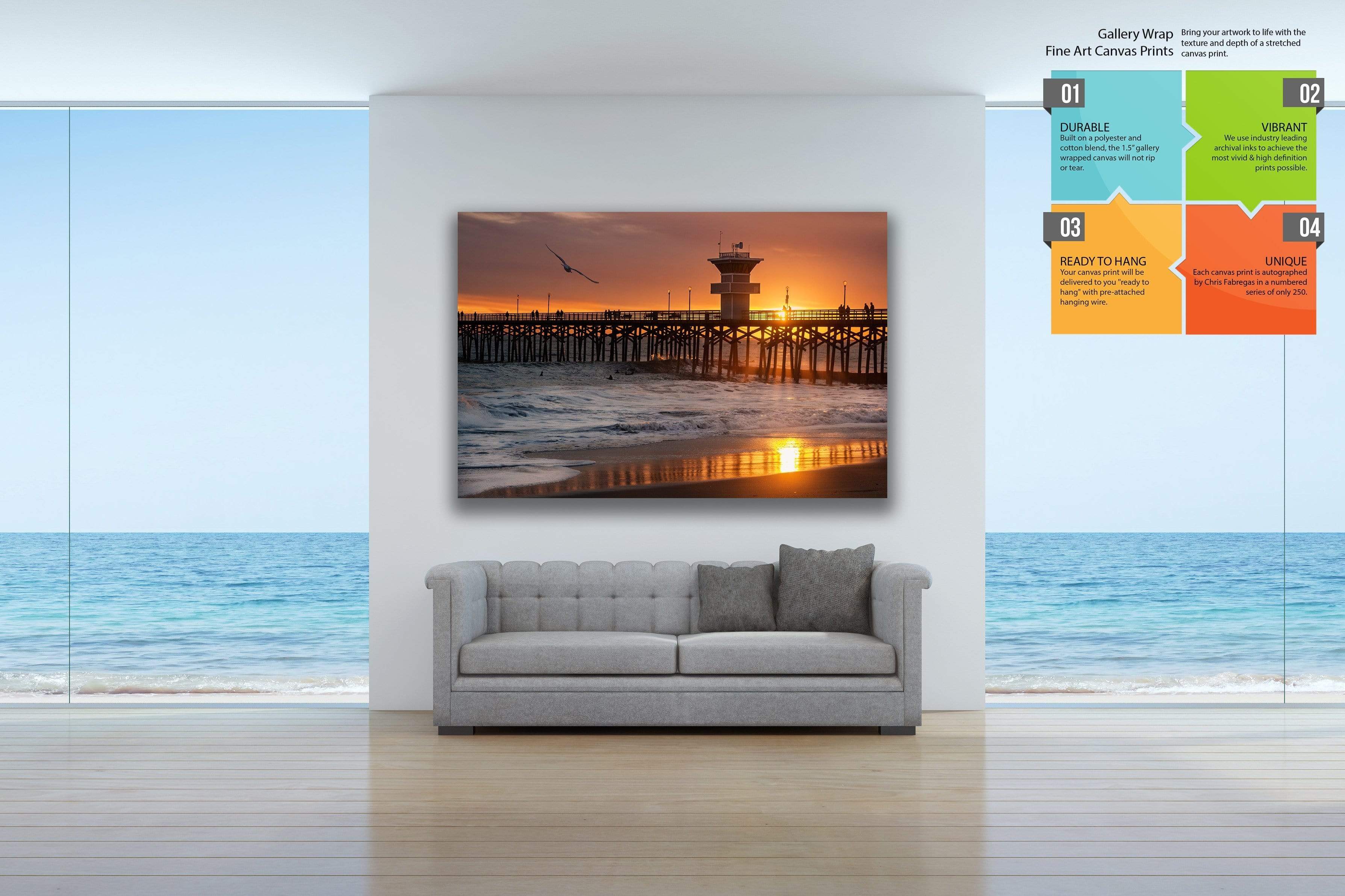This image captures the interior of a modern, seaside home with a breathtaking view of the ocean. Dominating the foreground is a light gray couch adorned with two darker gray pillows. The couch is positioned against a stark white wall, which splits the glass wall into thirds. Above the couch hangs a large, vivid photograph of a sunset at a beach pier, with a lighthouse or guardhouse and seagulls flying through the glowing sky. Both the left and right sides of the white wall are flanked by floor-to-ceiling glass windows, offering an unobstructed view of the ocean waves almost reaching up to the glass. The sun's reflection glimmers over the water, enhancing the serene atmosphere. The room features horizontal plank flooring that adds to its modern aesthetic. In the top right corner of the image, there's a multicolored infographic divided into blue, green, orange, and red sections, labeled Gallery, Wrap, Find, Achievements, and Prints, providing additional information about the artwork on display.